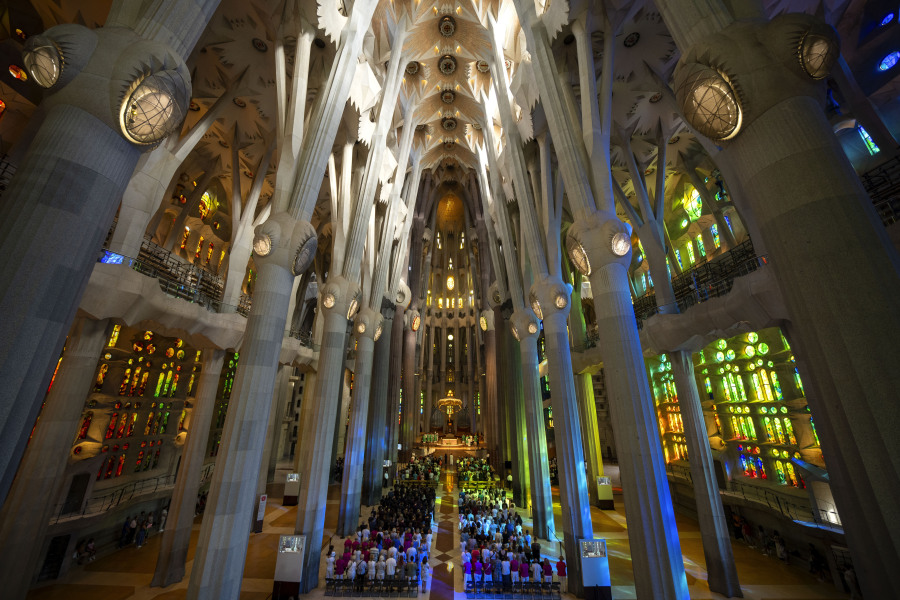This photograph captures the grandeur of a highly ornate and beautiful cathedral interior, characterized by its towering, marble-like white pillars that soar 40-50 feet into the air, supporting the vaulted ceilings. The walls are adorned with intricate details and feature stunning stained glass windows on both sides, predominantly in shades of red, blue, yellow, and green. These windows allow sunlight to cascade into the cathedral, illuminating the space with vibrant colors. The cathedral is filled with rows of pews, where a large congregation, dressed variably in reds, whites, pinks, and darker hues, is seated, engaged in prayer or other ceremonial activities. A long aisle runs down the middle of the room, leading to a somewhat out-of-focus setup, possibly including a pulpit or a statue, at the center of the pews. The circular lights hanging high above add to the majestic ambiance of the scene, encapsulating a moment of solemn reverence within this magnificent architectural marvel.